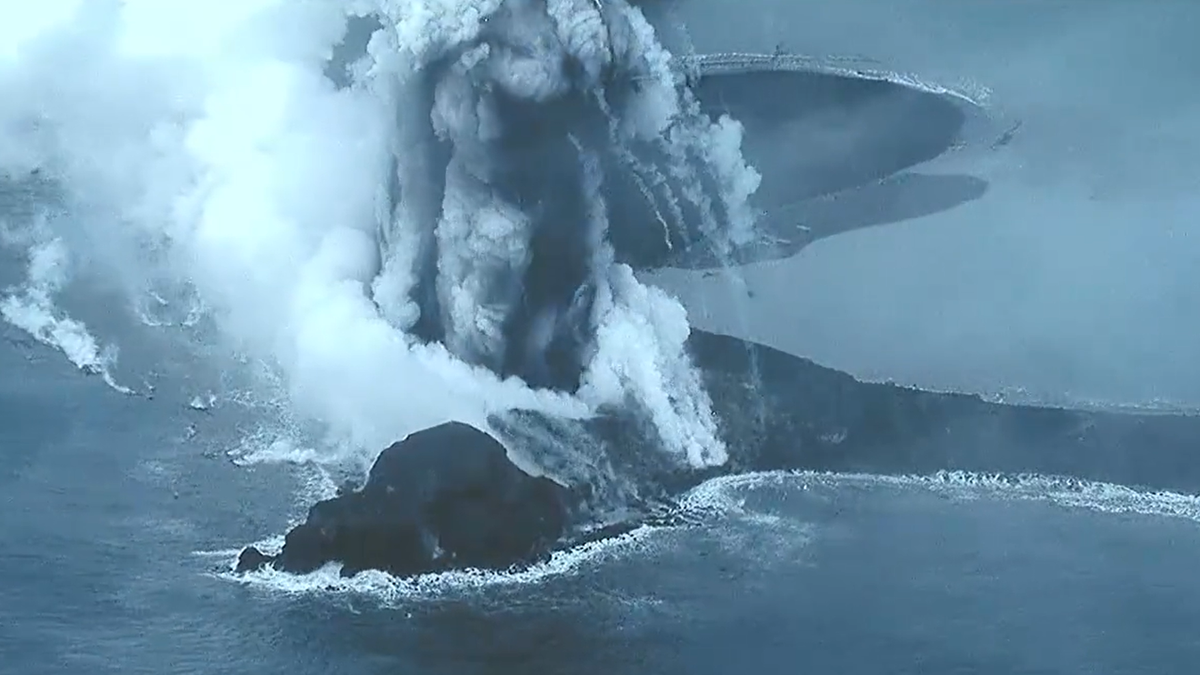This image presents an aerial view, possibly captured by a drone or helicopter, of a dramatic volcanic eruption occurring on a small island, likely situated in the middle of the ocean. The volcano, positioned near the base level of the ocean, is actively erupting, emitting massive plumes of dark gray and white smoke, ash, and steam. The surrounding landscape, a combination of black landmass and flat terrain, stretches horizontally and jets out towards the viewer, forming a picturesque yet foreboding scene. The sky above is filled with ominous gray clouds, enhancing the dramatic atmosphere of the eruption. The island appears uninhabited and of modest size, suggesting minimal damage despite the intensity of the eruption. In the background, a massive flatland is visible, contributing to the expansive and isolated feel of the scene.